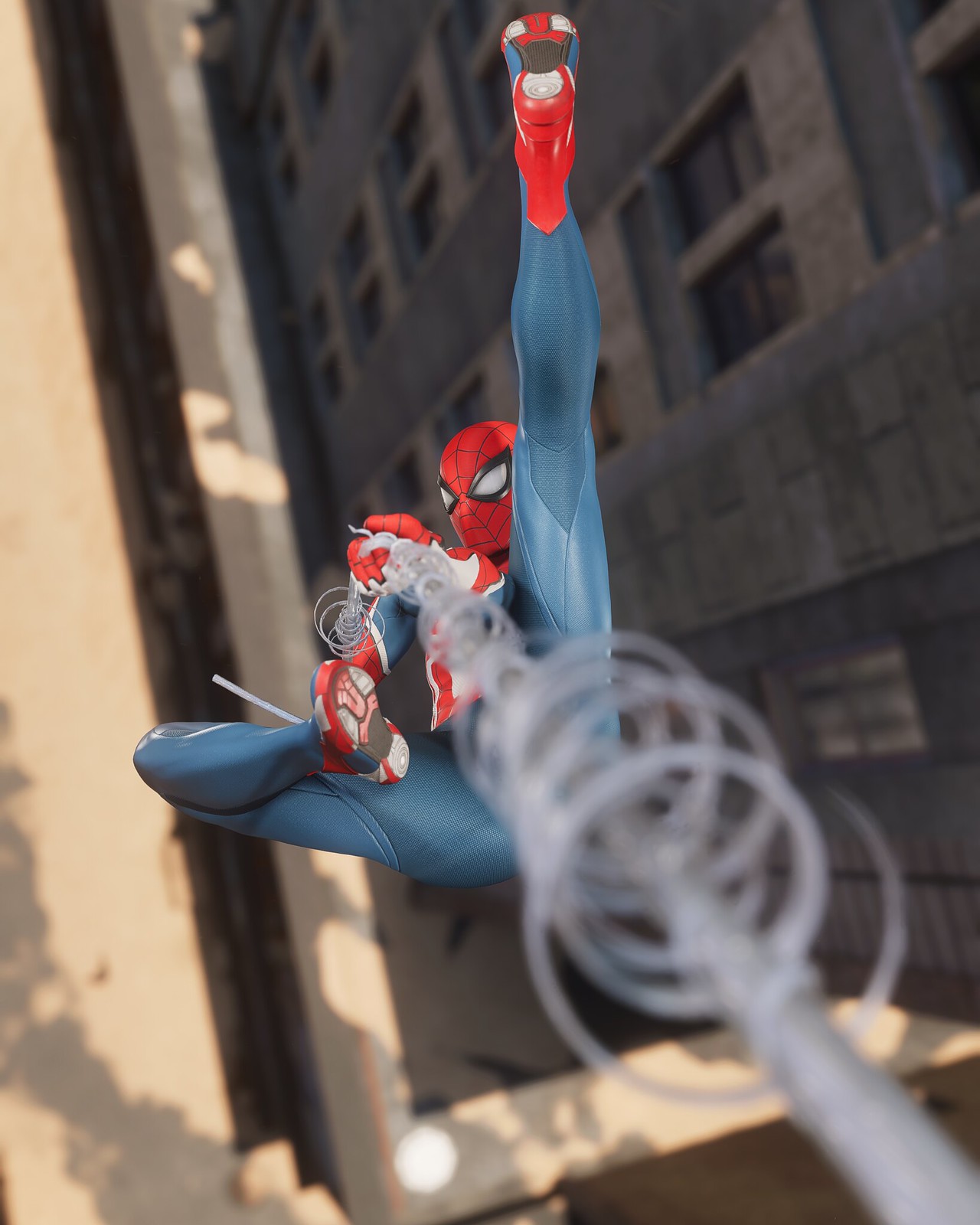The animated scene features Spider-Man centrally positioned, descending upside down from a light gray web that extends from the bottom right corner of the frame. The web itself is detailed with a cylindrical center and numerous smaller spiraling strands encircling it, creating a dynamic visual effect. Spider-Man's athletic pose is well-captured; his left leg extends upwards toward the top left of the image, while his right leg bends at the knee, forming a triangle. This positioning partially obscures his iconic masked face behind his outstretched left leg. The vibrancy and detail suggest a polished rendering, likely from a movie or a high-quality video game.